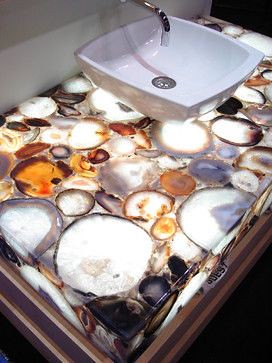This photograph captures a stunning bathroom countertop, artistically designed for a bathing area. The countertop, likely crafted from acrylic, features an array of oceanic shells embedded within it, creating a captivating, seaside aesthetic. The transparent acrylic surface, thick and sturdy, showcases various types of shells, including broad, bubble-like specimens, enhancing its visual appeal.

A white, surface-mounted sink is centrally positioned atop this decorative acrylic countertop. A chrome or stainless steel drain is seamlessly integrated, with a faucet spout elegantly extending from the wall above the sink. Although the faucet knobs are not visible in this image, they are presumably situated just above the cropped upper edge of the photo. Supporting the countertop is a cabinet or set of support legs, ensuring stability and functionality. The backdrop of the scene features a sleek, gray wall, complementing the modern and artistic design of the bathroom.